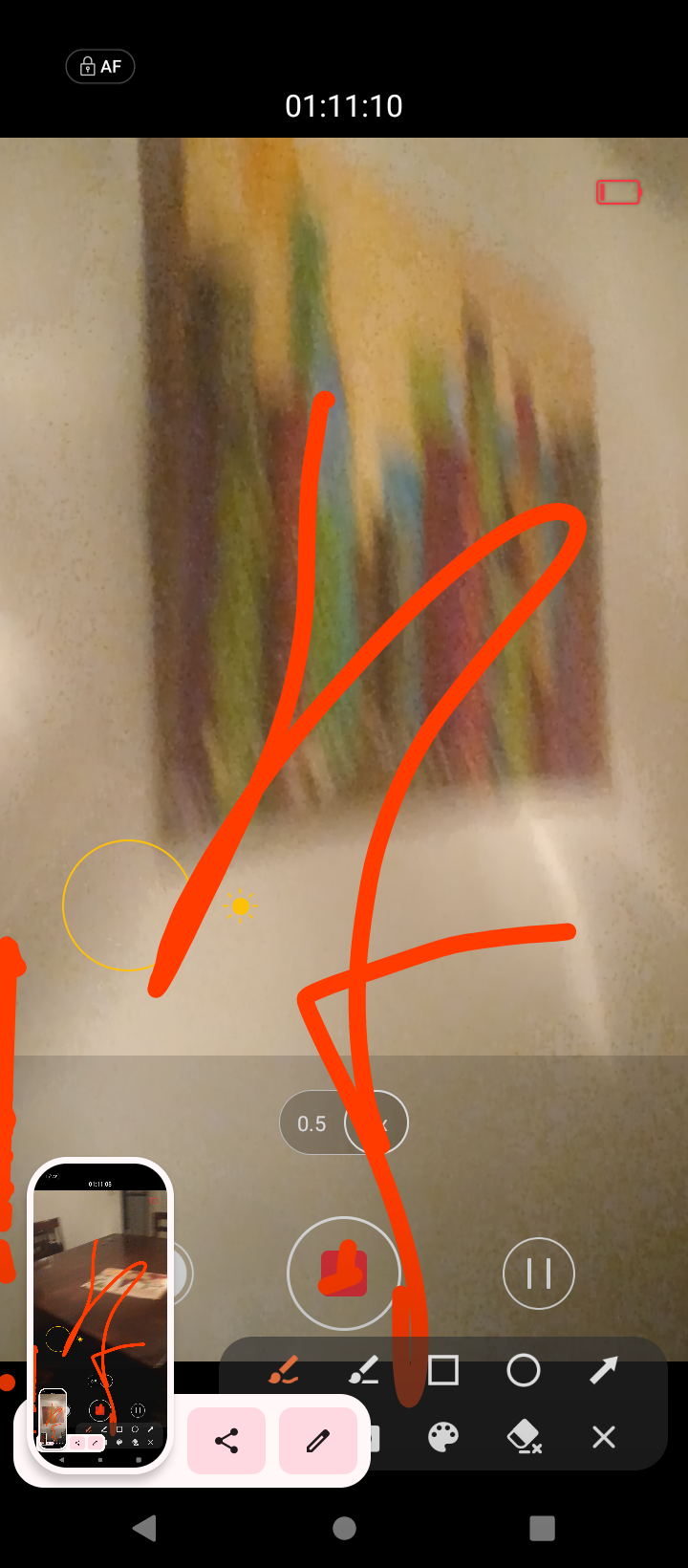In this image, a blurry screenshot of a phone's screen is shown, which is being edited using the phone's markup tool. A black banner spans the top of the screen, displaying "AF" followed by the time, 01:11.10. The battery icon is nearly depleted, indicating low battery life. In the screenshot, a blurred painting is visible hanging on a wall. A prominent red scribble, created using the marker tool, is drawn in the middle of the image. At the bottom of the screen, the editing tools are actively open, revealing options such as a 0.5x zoom level and a pause button. The overall scene suggests someone is in the process of annotating or altering the image using basic image editing functionalities on their smartphone.